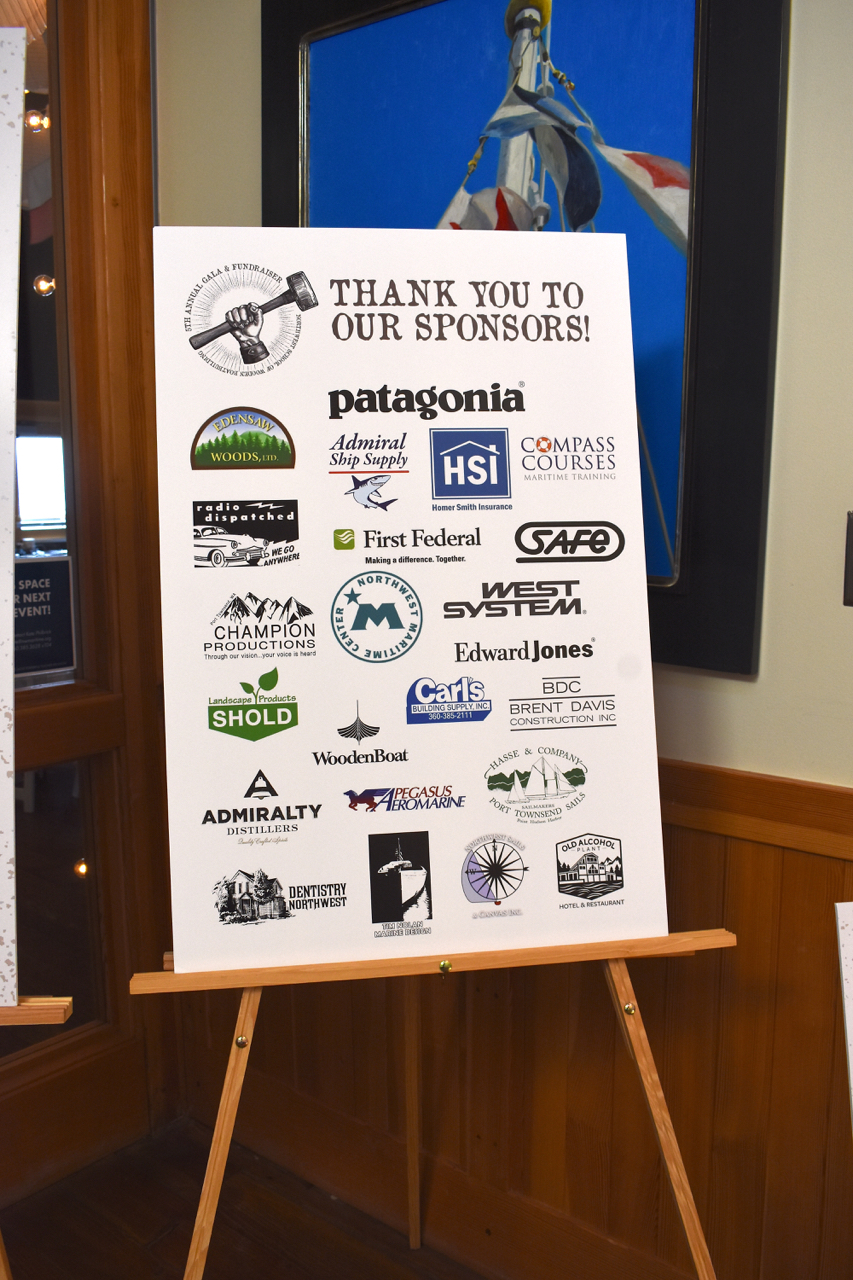This photograph depicts a light wooden easel holding a white poster board prominently displaying a "Thank You to Our Sponsors" message, along with an array of corporate logos. Noteworthy sponsors include Patagonia, Schold, West System, Edward Jones, Wooden Boat, Admiral Ship Supply, HSI, Compass Courses, First Federal, SAFE, Champion Production, Carls, BDC, Brent Davis, Construction Income, Admiralty, Dentistry Northwest, and Old Alcohol. The poster board features an image of a hand holding a gavel at the top and is placed within a room that appears to be a conference center, characterized by wood paneling on the walls. Behind the poster, there's a framed picture of an American flag with a blue background, partially obstructed by the easel.